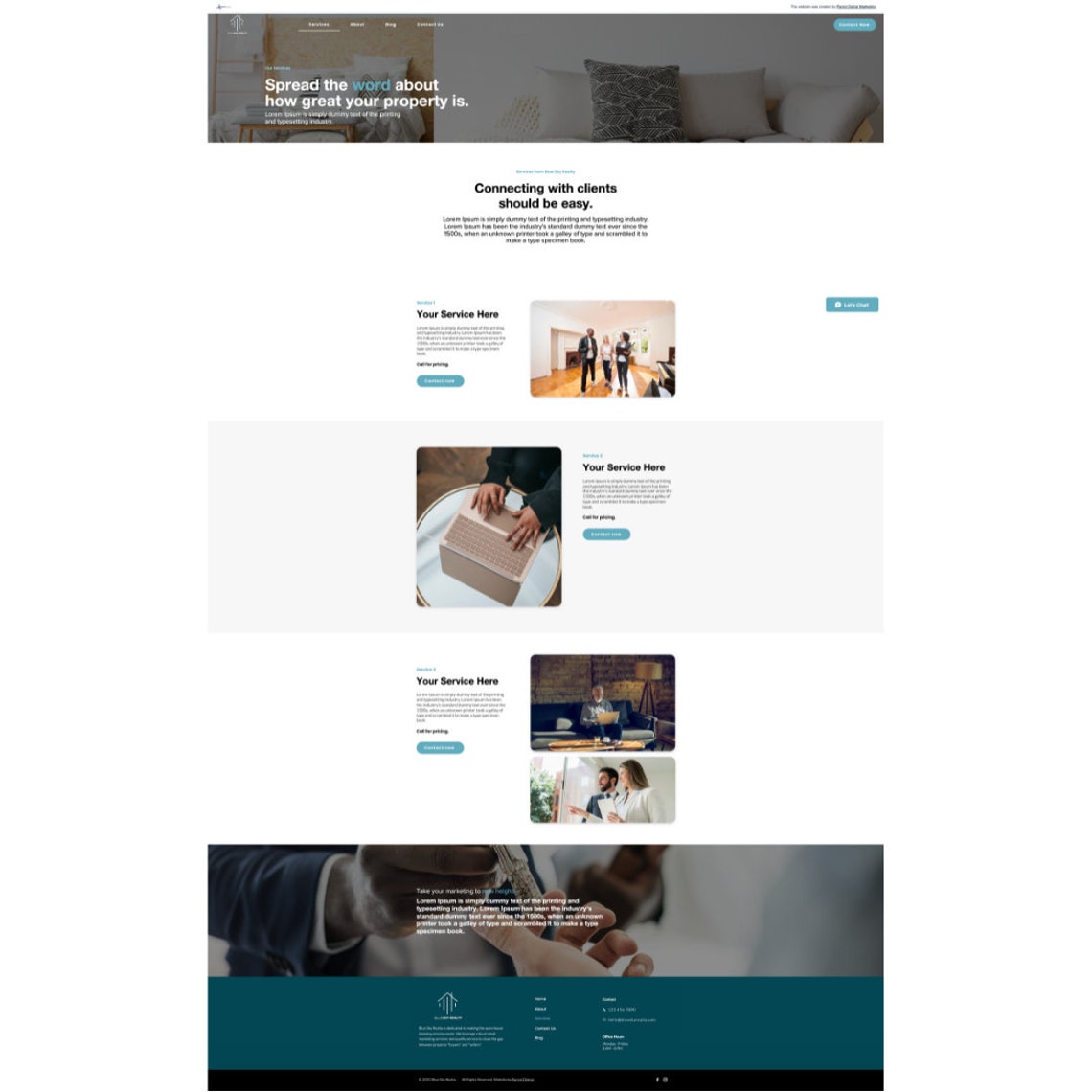The image is a screenshot from a webpage that features a promotional banner at the top. Despite some blurriness, the banner prominently displays an assortment of pillows arranged on either a couch or a bed. The text "Spread the word about how great your property is" is displayed, with the word "word" uniquely highlighted in teal while the rest of the text is in white. Below the banner, there's a section titled "Connecting with clients should be easy" accompanied by a small paragraph of text. 

Further down, an image features three people standing together near the top middle of the webpage, with the text "Your service here" positioned nearby. Another picture shows a woman with her hands on an object, also captioned "Your service here." Both these sections include teal-colored buttons that, when clicked, provide more information.

At the bottom of the webpage, contact information and other relevant details are listed, concluding the content of the page.